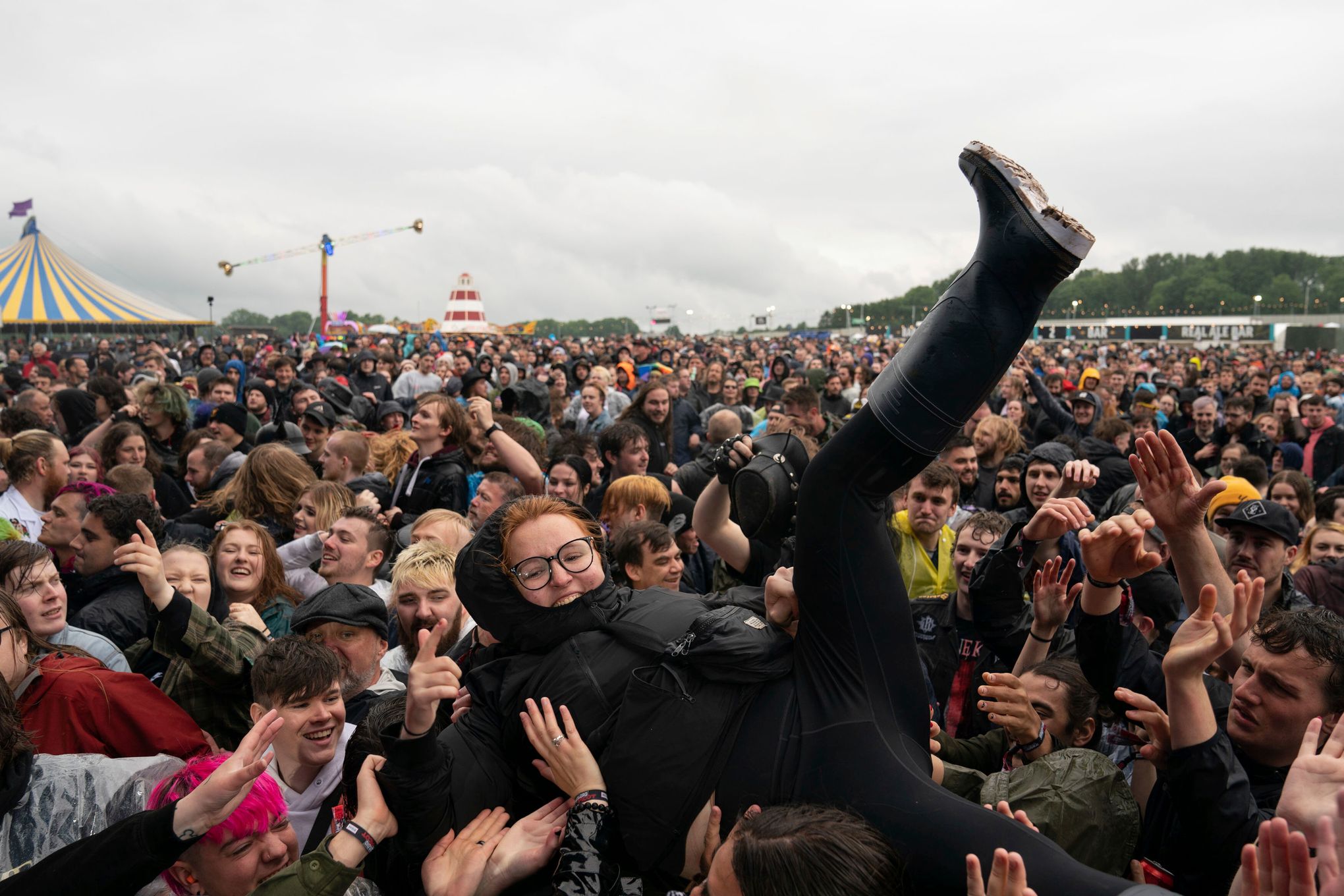The image captures a bustling outdoor fair or celebration with a massive crowd of people having a great time. Colorful, circus-like tents and several amusement park rides dot the background, reminiscent of attractions you might find at a place like Six Flags. In the foreground, a young woman with reddish-brown hair, wearing a black hooded coat, black pants, and black boots, is being crowd-surfed. She has black-framed glasses and a black pouch hanging in front. A sea of hands hoists her up, and smiles abound as people enjoy the festive atmosphere. The expansive crowd suggests a popular event, with countless individuals relishing the entertainment and camaraderie.